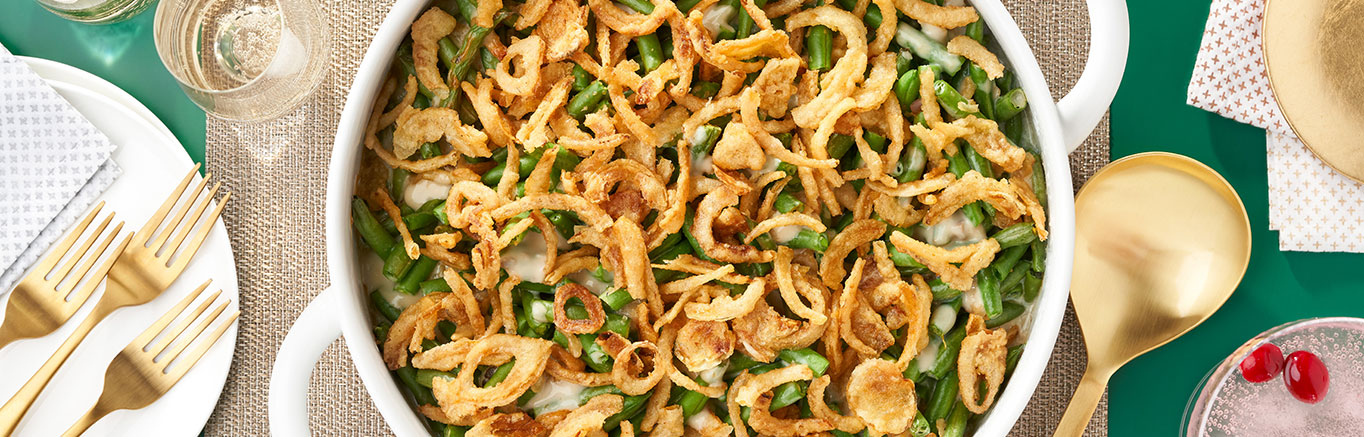This indoor photograph, rectangular in shape and approximately six inches wide by one and a half inches high, provides an overhead view of a meal setting centered around a large white bowl filled with green bean casserole. The casserole features long green beans smothered in a creamy white sauce, topped with crispy, golden-brown fried onions. The white dish extends off the top and bottom of the image, resting on a light brown canvas placemat atop a green table. 

To the upper left of the bowl, there's a clear glass filled with a bubbling clear liquid, possibly water. In the lower left, a white plate holds three golden forks alongside star-printed napkins. 

On the lower right side, another glass containing a clear fizzy drink with two maraschino cherries can be seen. Adjacent to this is a gold-colored spoon. The upper right corner features white napkins with gold X's partially covering a gold-colored plate, adding a touch of elegance to the setting. This detailed arrangement evokes a celebratory or holiday meal atmosphere, reminiscent of Thanksgiving dinners.